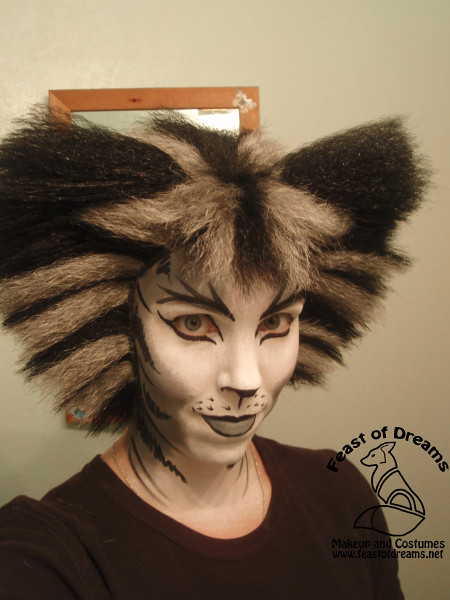The image features a young woman who has meticulously applied makeup to resemble a performer from the musical "Cats." Her face is painted white with detailed gray shading on her cheeks, creating a shadow effect near her mouth. She added speckled dots above her lips to signify whiskers, and her lips are painted gray with a black outline. A black patch under her nose mimics a cat's nose. She has black stripes on her eyebrows and cat-eye makeup, along with striped patterns on her cheeks similar to a tabby cat. She is also wearing a black and white wig styled to resemble cat ears, reminiscent of the wigs worn by characters in "Cats." The woman exudes confidence as she looks at the camera, dressed in a simple black shirt. In the background, there is a light-colored wall and a wooden-framed mirror. The bottom right corner of the image features a watermark with a fox logo and text that reads, “Feast of Dreams, Makeup and Costumes,” with the website "FeastofDreams.net."